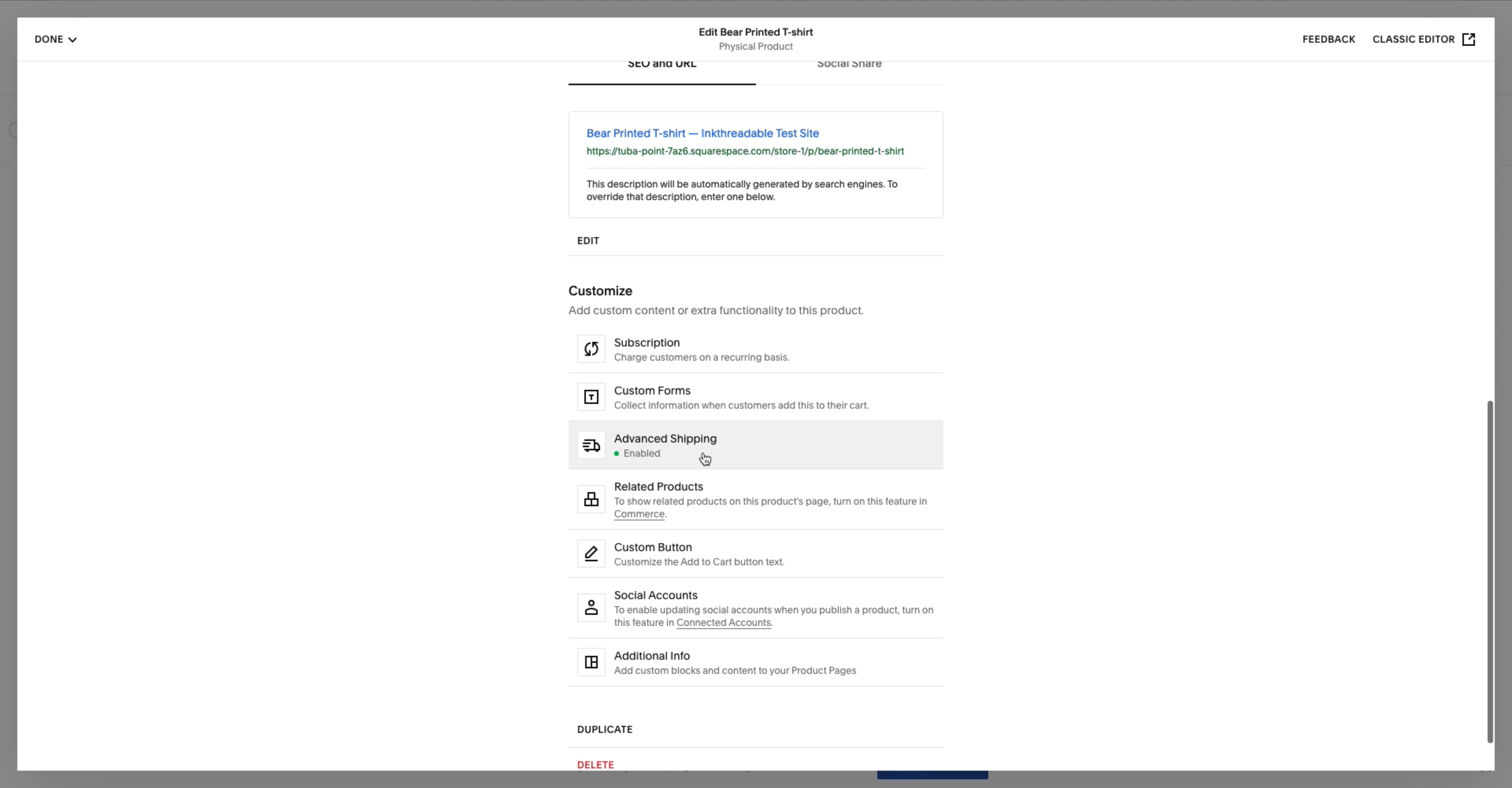Screenshot of an e-commerce customization tool webpage with white background. The page lacks any identifiable company branding, header, or footer. In the center, a gray font headline states, "Edit a Bear Printed T-Shirt." Below this, in standard text, it reads "Physical Product," followed by a blue text label, "Bear Printed T-Shirt." There is partially readable text indicating "Test Site," suggesting this may be a developmental or preview mode of the tool. The page features a list of customization options including "Subscription," "Custom Forms," and "Advanced Shipping." This utility page appears designed for e-commerce website owners to tailor their product listings and shipping options.